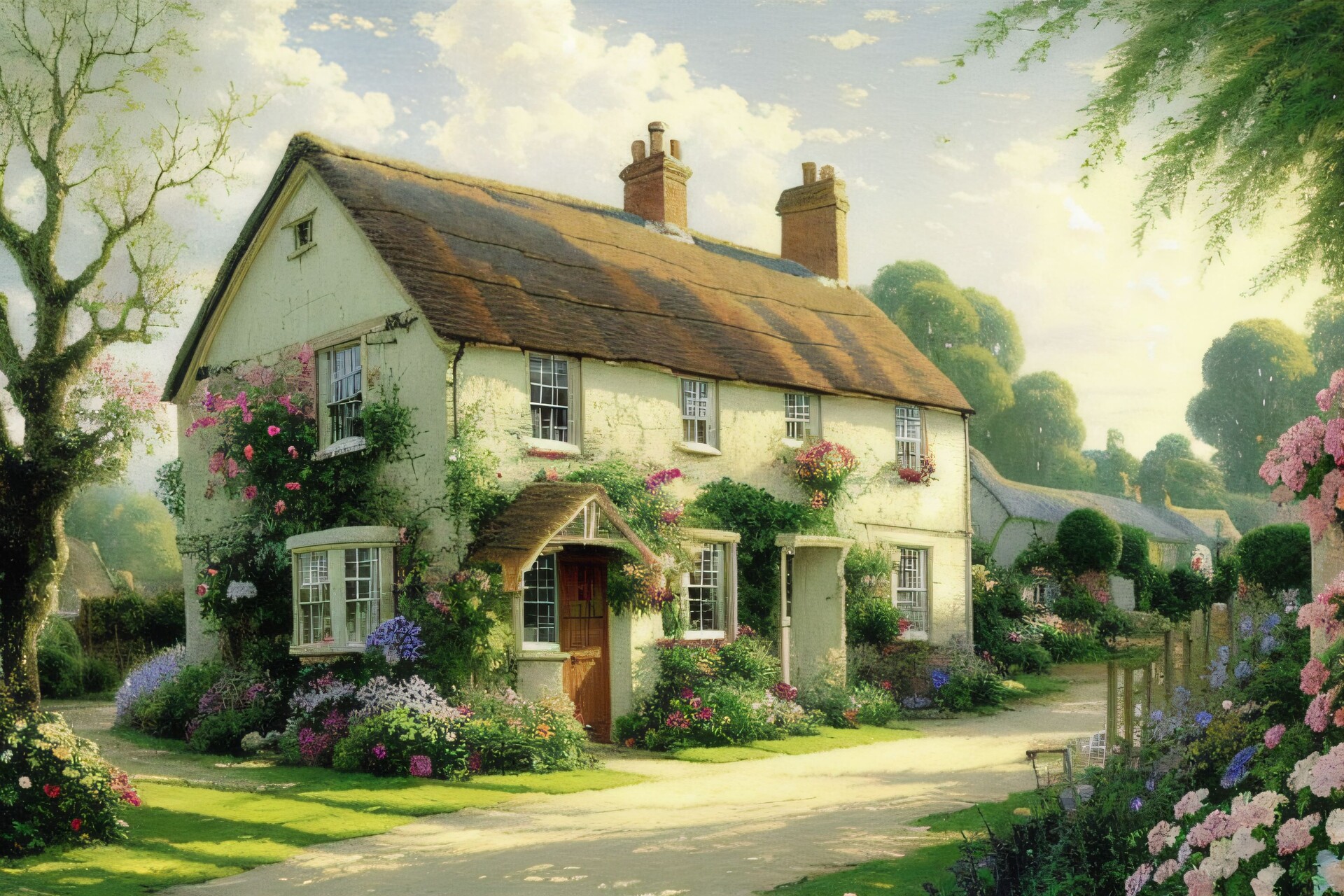The image depicts a detailed, softly focused painting in the style of Thomas Kinkade, showcasing a serene outdoor setting during the daytime. The focal point is a charming two-story English country cottage with a white exterior, accentuated by a red, gabled, steeply pitched roof, adorned with two chimneys, each adorned with three spouts. The house is presented in a three-quarter view, allowing an engaging look at its defining features, including the prominent gabled roof over the entryway and a bay window on the side, both embellished with pristine white frames.

Clusters of climbing roses with pink flowers and white flowering bushes grace the sides of the house, adding a vibrant palette of pastel colors. The right side of the image, along the bottom, features a flower bush with light pink tones and green leaves, extending slightly out of frame. A picturesque dirt road, light in color, curves from the bottom left to the middle right, leading to the house. This road is bathed in sunlight, complemented by the blue sky and scattered white clouds above.

Surrounding the house, the landscape is lush with various flowering bushes and a tall, leafless tree with lower branches adorned with tiny blossoms, enhancing the tranquil, pastoral ambiance. The foreground includes a set of stones upright on the lawn, providing a rustic touch.

In the distance, another building emerges, partially hidden but framed by neatly trimmed shrubs. The background features the leafy tops of additional green trees, completing the idyllic countryside scene.